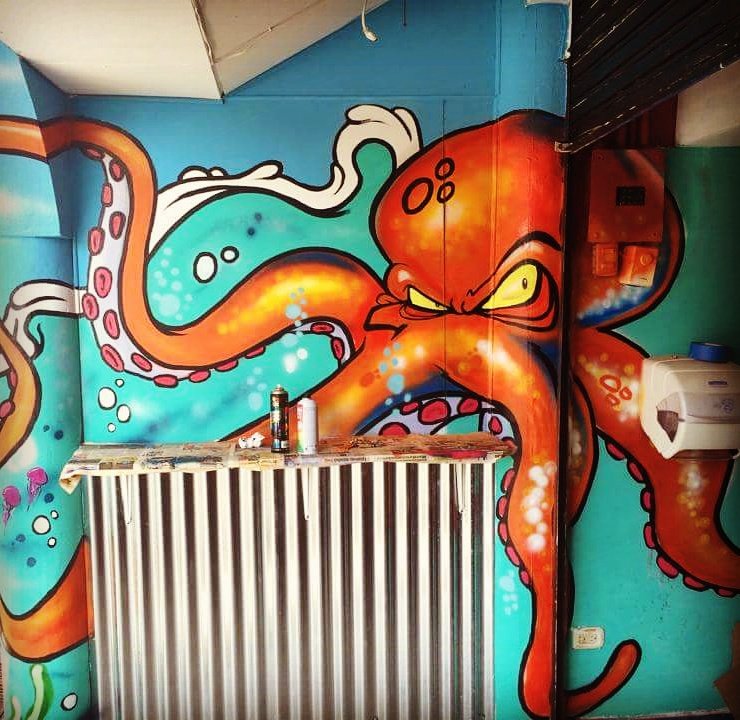The image depicts a vibrant and unique mural spray-painted on a blue wall, possibly within a bathroom setting suggested by the presence of a hand towel dispenser on the right side of the wall and a radiator-like vent near the center. The mural features a striking, cartoonish octopus with a large, round, red-orange head and mean-looking, furrowed yellow eyes staring to the right. The octopus’s tentacles display detailed suckers in shades of pink and light blue, with teal and turquoise tonal variations underneath, contributing to the aquatic atmosphere. Surrounding the octopus is a dynamic water depiction with turquoise tones, light blue bubbles, and cartoonish white splashes. To the left of the mural, there is a section covered in newspaper, suggesting an area used for spray-paint artwork, complete with spray paint cans and a little table with scattered paper, likely to catch any paint drizzles.